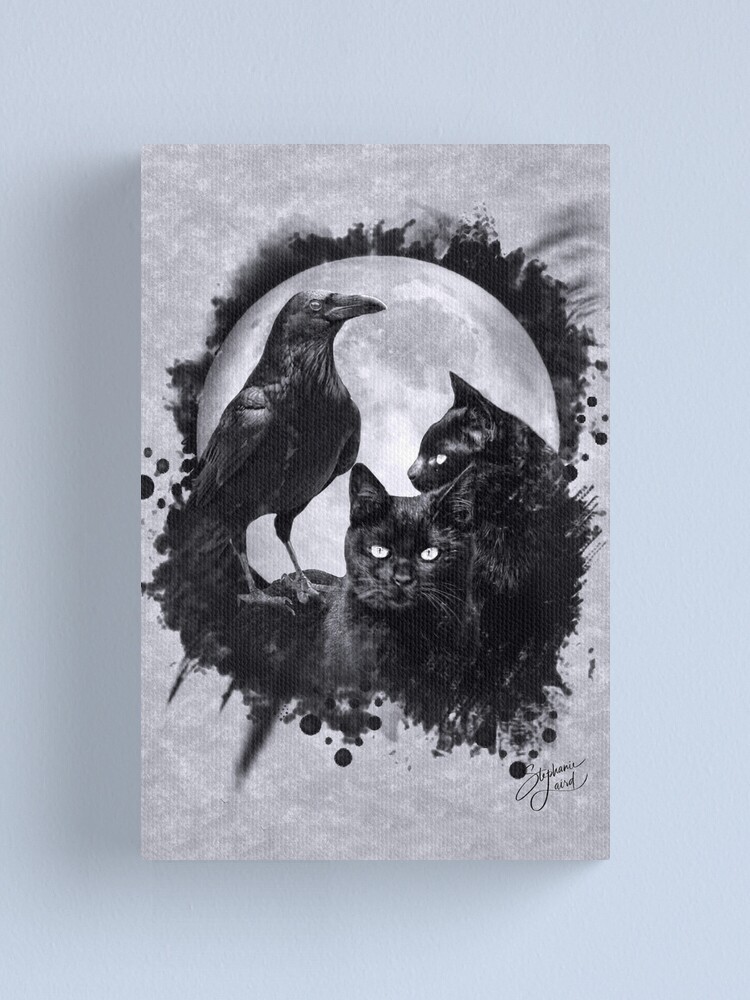This image appears to be a highly detailed charcoal painting featuring a black crow and two black cats set against an intricate backdrop of silver-gray and black tones. The background has a charcoal-like texture with varying shades of gray and white, highlighting the very dark and moody atmosphere of the scene. At the top center of the image, there is a black moon with a splash-like aura radiating outward, adding an eerie glow. The black crow is perched prominently in the middle, gazing to the right. Around it, the first black cat, positioned at 3 o'clock, faces left while the second one, situated at 6 o'clock, stares straight ahead with very large, seemingly angry eyes. The animals appear clustered together as if part of a dark celestial narrative. The piece is signed "Stephanie" in the bottom right corner, though the script is somewhat difficult to decipher. The entire composition is rendered in a stark monochrome palette, amplifying the dramatic and mysterious tone of the artwork.